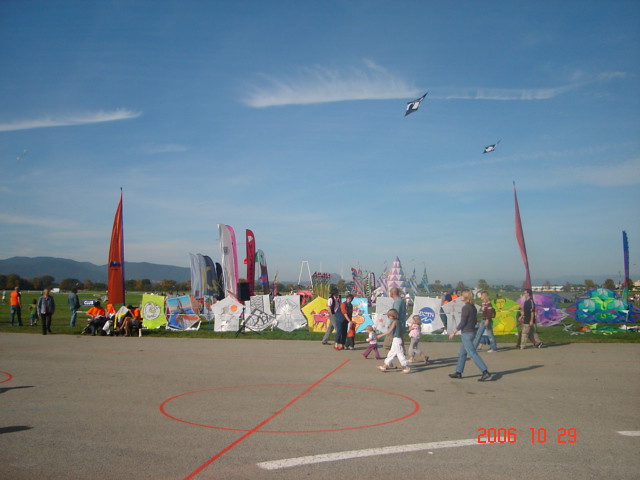The photograph captures a vibrant kite flying event taking place on a bright and sunny day, with a timestamp indicating it was taken on October 29, 2006. The scene is set on a spacious area of pavement with distinct sports markings, resembling a basketball or football court, highlighted by red and white lines and a semi-circle. Numerous colorful kites are displayed on the ground, with a couple visibly soaring in the clear blue sky that features some wispy clouds. In the foreground, a family walks across the concrete, and other people, some wearing orange t-shirts, parade around or sit on the grass beyond the pavement, indicating a lively atmosphere with spectators on both the concrete and grassy areas. Tall kites, possibly used for kite surfing, along with umbrellas positioned in the background, add to the festive ambiance of this outdoor event.